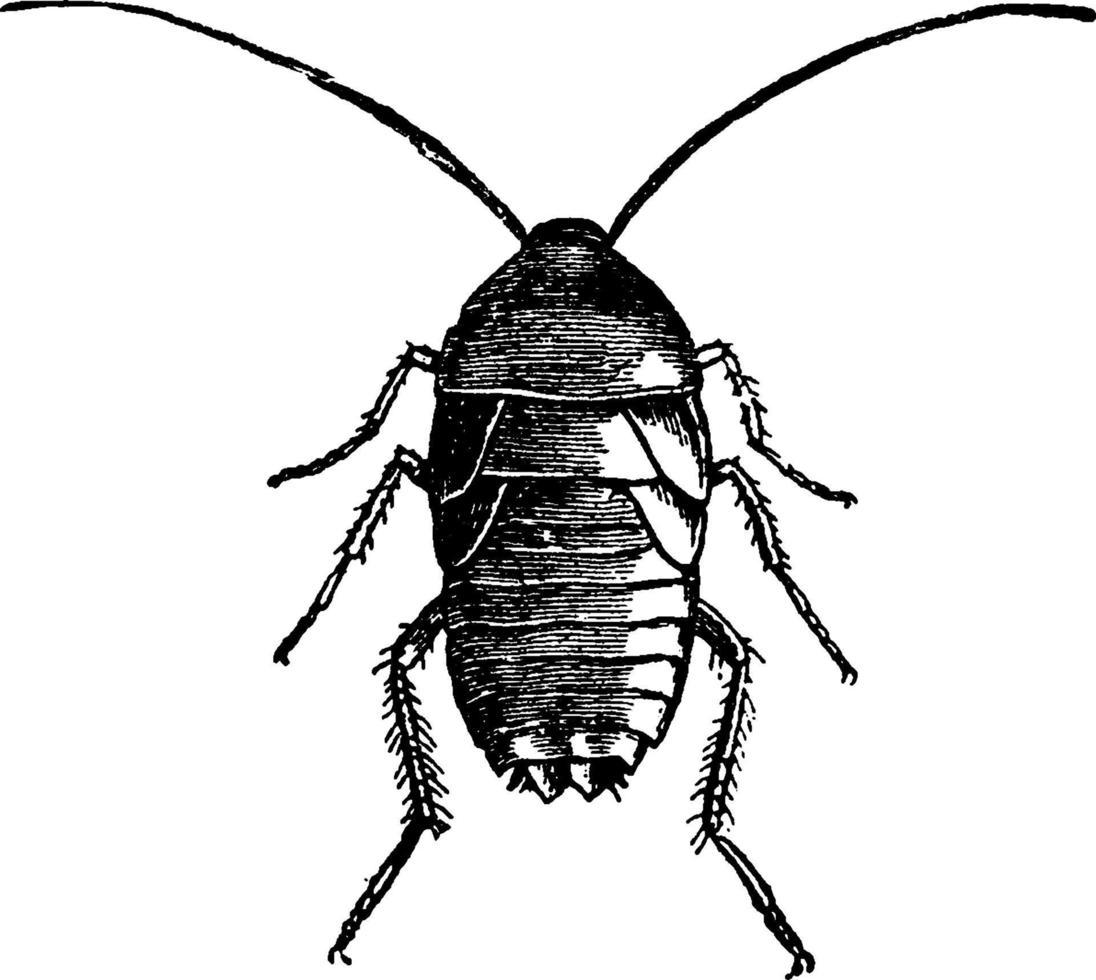This detailed black and white drawing captures a top-view silhouette of a large, segmented insect resembling a cockroach or beetle. The meticulously sketched image showcases two prominent antennae extending approximately four inches each, curving outward from the head towards the upper corners of the drawing. The insect's six legs, three on each side, are depicted with fine lines representing tiny hairs, giving a textured, scaly appearance. The body of the insect is broad and flat, adorned with horizontal and vertical scales. These scales are predominantly white with black lines, adding to the depth and detailed shading of the sketch. The insect's rear end tapers into two pointed, inverted triangles. Set against a stark white background, the image features distinct shading techniques, emphasizing the intricate details like the scales and fur on the legs, making the drawing both precise and artistically shaded.